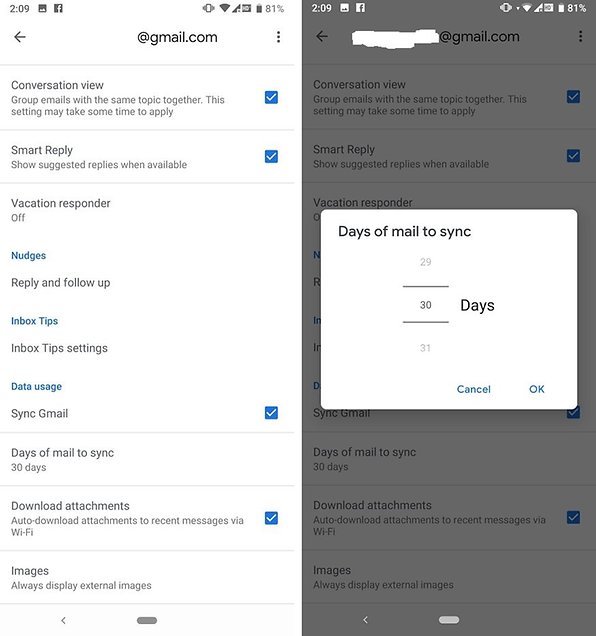The image is an amalgamation of two smartphone screenshots, focusing on email settings within a Gmail account. Starting from the top, both screenshots display the typical smartphone indicators in grey, such as battery percentage and Wi-Fi connectivity. They also feature a back arrow and an "@gmail.com" address at the top, signifying the account in use.

The main screenshot outlines various configurable settings, each accompanied by checkboxes. The first setting, labeled "Conversation view," with a grey description stating, "Group emails with the same topic together. This setting may take some time to apply," is enabled as indicated by a blue checkmark. The "Smart reply" option, designed to show suggested replies when available, is also active with a blue checkmark beside it. 

Further down, the "Vacation responder" is noted to be off, while "Nudges," "Reply and follow up," "Inbox tips," and "Inbox tip settings" are listed without explicit activation status. 

Under "Data usage," it mentions syncing Gmail with a blue checkbox indicating it is enabled. Linked to this is the "Days of mail to sync" setting, currently set to 30 days. Following this, the "Download attachments" option, which auto-downloads attachments in recent messages via Wi-Fi, is checked in blue. Lastly, the setting for "Images," which always displays external images, is enabled.

The second screenshot mirrors the same settings as the first but includes a pop-up dialog box titled "Days of mail to sync." It lists various options for the number of days to sync mail, with 30 days highlighted as the current selection. This dialog box features two buttons at the bottom: a blue "Cancel" button and a blue "OK" button, both set against a white background with black text, allowing the user to confirm or cancel any changes to this setting.